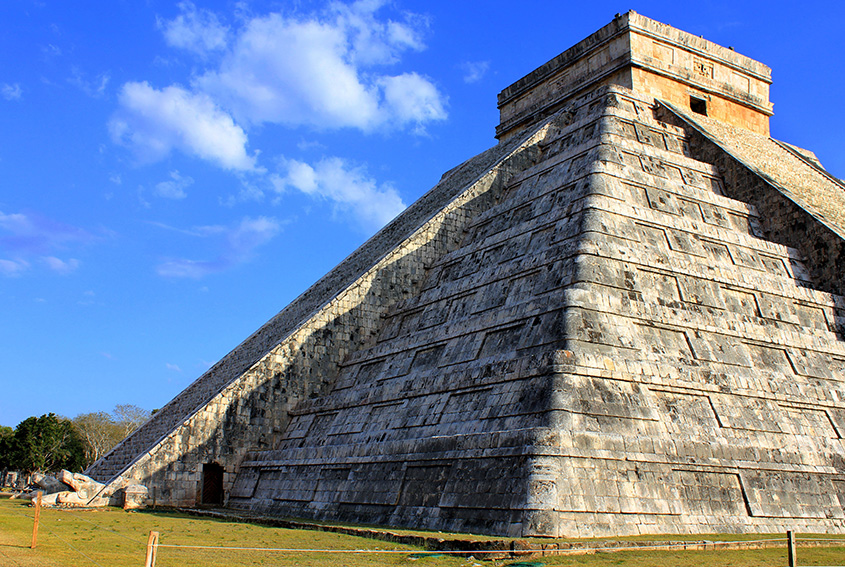This photograph, taken outdoors on a bright, sunny day with a blue sky and white clouds, features an ancient Mesoamerican pyramid prominently in the center-right. Judging by its architectural style, characterized by its multiple terraced steps climbing steeply to the top and constructed from dark gray and white square stones, the pyramid appears to be of Mayan or Aztec origin. The pyramid features two visible staircases—one on the left side near a clearly defined doorway and another on the right side—both leading up to a small temple entrance at the summit. Surrounding the base of the structure, there is a series of wooden stakes and wire, suggesting restricted access to prevent visitors from entering. Additionally, there seems to be a ditch or moat-like formation circling the pyramid, adding to the ancient and fortified impression of the site. The foreground features grassy terrain, while the background is lush with trees, enriching the historical and natural ambiance of the scene.